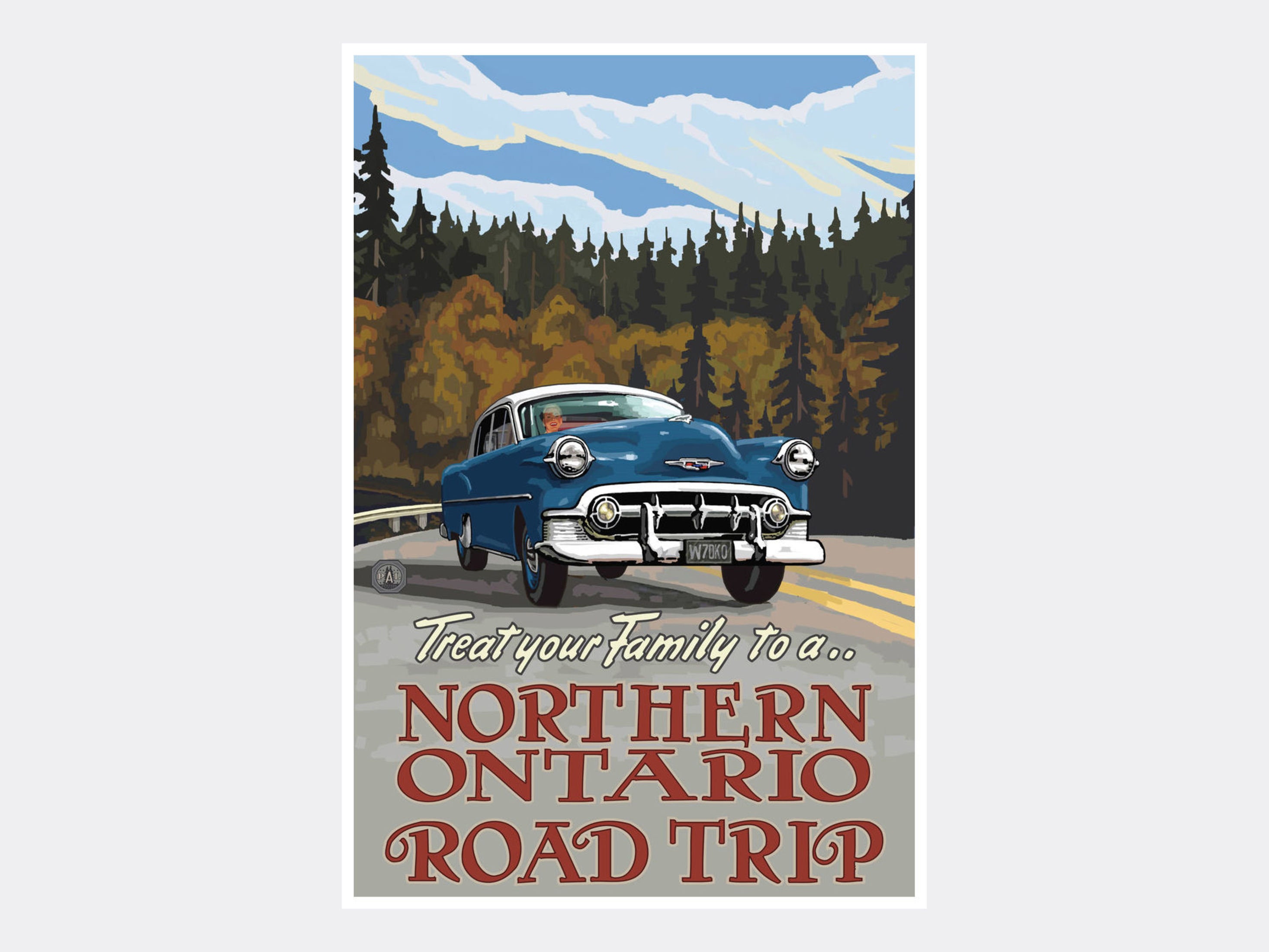The image features a high-quality, full-color lithograph poster from the 1950s era, depicting a classic blue Chevrolet on a winding road in northern Ontario. The text at the bottom reads "Treat your family to a northern Ontario road trip" in an interesting red font, with "Treat your family to a" in white italic letters with a black outline. The scene portrays the car, possibly a 50s-era sedan with the license plate starting with a 'W' and containing '7010', climbing a road adorned with a guardrail and leading towards the viewer. In the background, there is a lush forest of green conifer and lighter hardwood trees under a blue sky with light blue clouds. Vaguely visible are people in the car, suggesting a family outing. This visually appealing and collectible poster evokes nostalgia and promotes the allure of a scenic family road trip through Northern Ontario.